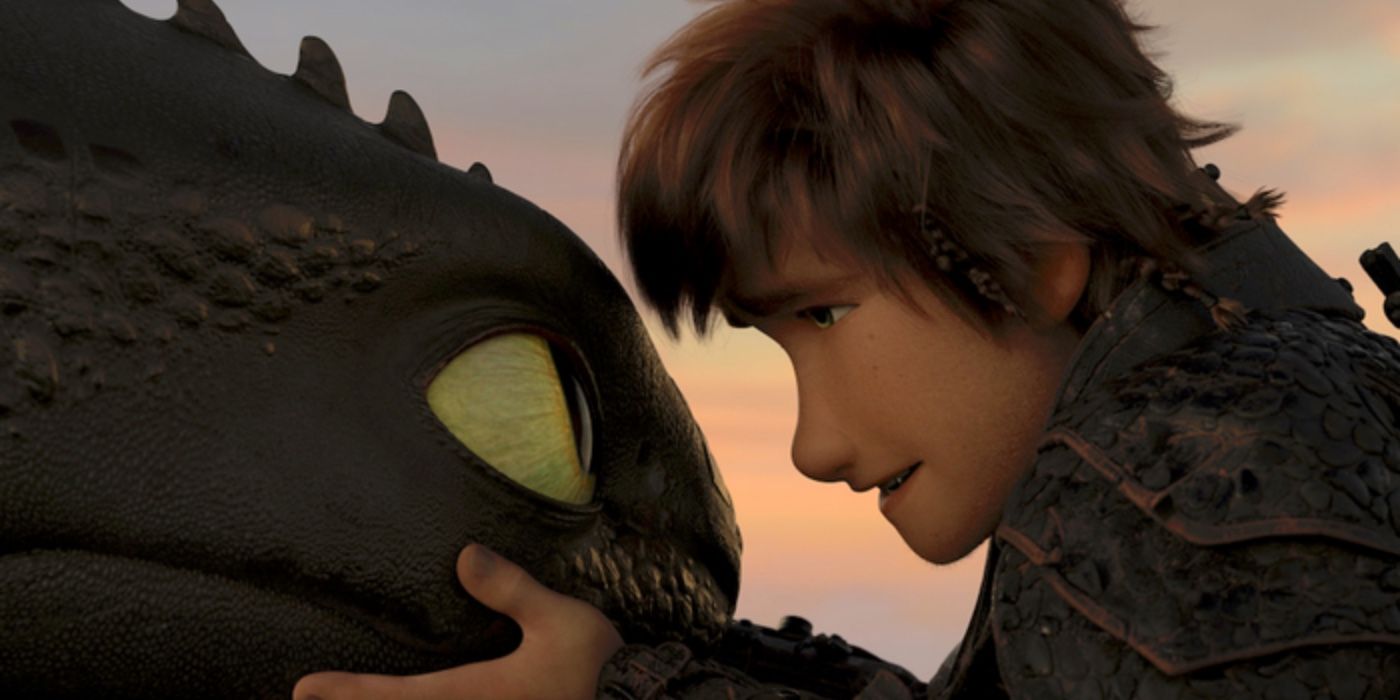The image is a still from one of the "How to Train Your Dragon" movies, depicting a poignant moment between a young boy and his dragon. The scene is animated in a 3D style, with the characters positioned in the center of the frame. To the left stands Toothless, the black dragon known for his sleek, almost reptilian appearance, with greenish-yellow eyes and distinctive spikes or fins on his head. Toothless is gazing up at his trainer, the boy standing to the right. The boy, identifiable as Hiccup, has brown hair, with several braids woven through it, and is shown in profile. He is clad in armor and is tenderly holding Toothless's face with his left hand, appearing to speak to the dragon. The background showcases a vibrant sky painted with hues of blue, pink, teal, and purple, suggesting a sunset in a fantastical realm.